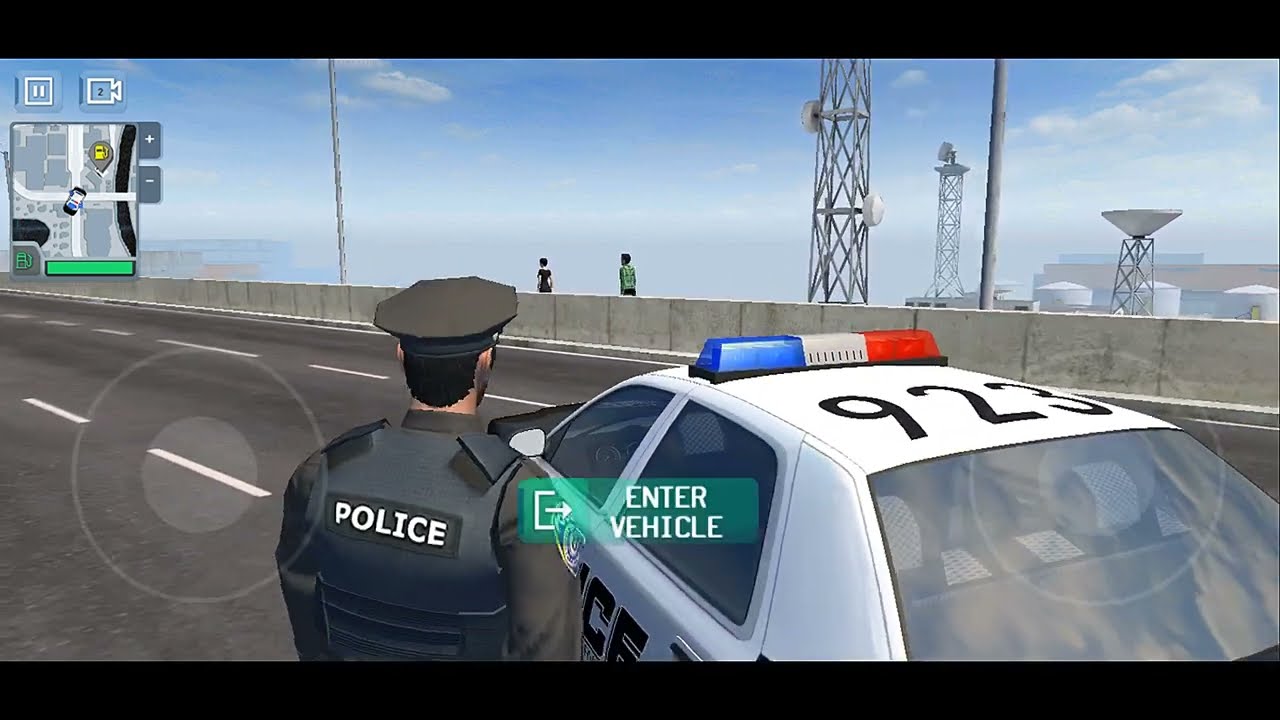The image is a detailed screenshot from a mobile video game, depicting a vivid urban environment filled with various elements. Central to the scene is a 3D model of a policeman dressed in a gray uniform and a bulletproof vest with "POLICE" written across the back, standing next to a black and white American police car marked with the number "923" on its roof and equipped with red and blue lights.

The setting is a three-lane road on a bridge, bordered by a concrete wall or barrier, and a few pedestrians can be seen walking along the other side. Visible in the distance are several metal towers adorned with satellite dishes and long silos, contributing to the urban-industrial backdrop. The sky is a clear blue, indicating a daytime scene.

Overlay features suggest it is a touchscreen game, with semi-transparent joystick circles on both sides of the screen. In the upper left corner, there is an in-game mini-map displaying a crossroads, a police car icon, and buildings along with pause and camera icons. At the center, a light green, transparent rectangle prompts the player with "Enter Vehicle" in white text, featuring an icon of a rectangle with an arrow pointing right. The road itself has distinctly marked white lane separators, further enhancing the realistic detail of the game environment.